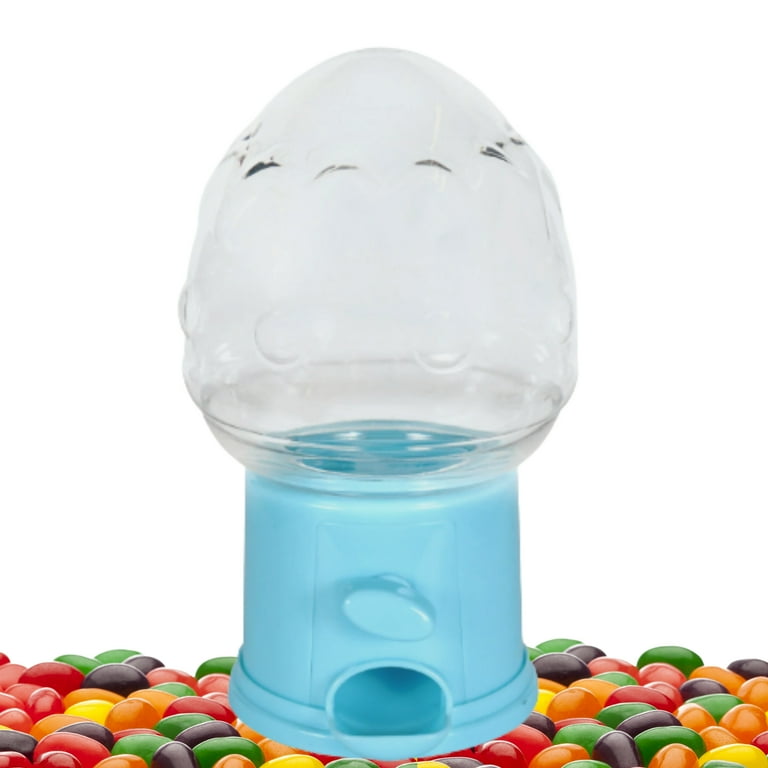The photo depicts a small toy gumball machine with a blue plastic base and a clear plastic dome. The dome, shaped somewhat like an inverted pinecone, is empty, indicating that no gumballs are inside. The gumball machine sits on a bed of colorful jelly beans scattered across the horizontal surface in front of it. The jelly beans come in various colors including red, yellow, orange, green, purple, and darker hues possibly resembling licorice flavor. The background behind the gumball machine and jelly beans is completely white, with no additional context provided. The overall appearance suggests that the machine is more for display or storage than actual use, as it lacks a heavy-duty metal turner and doesn't appear to have a coin slot mechanism.